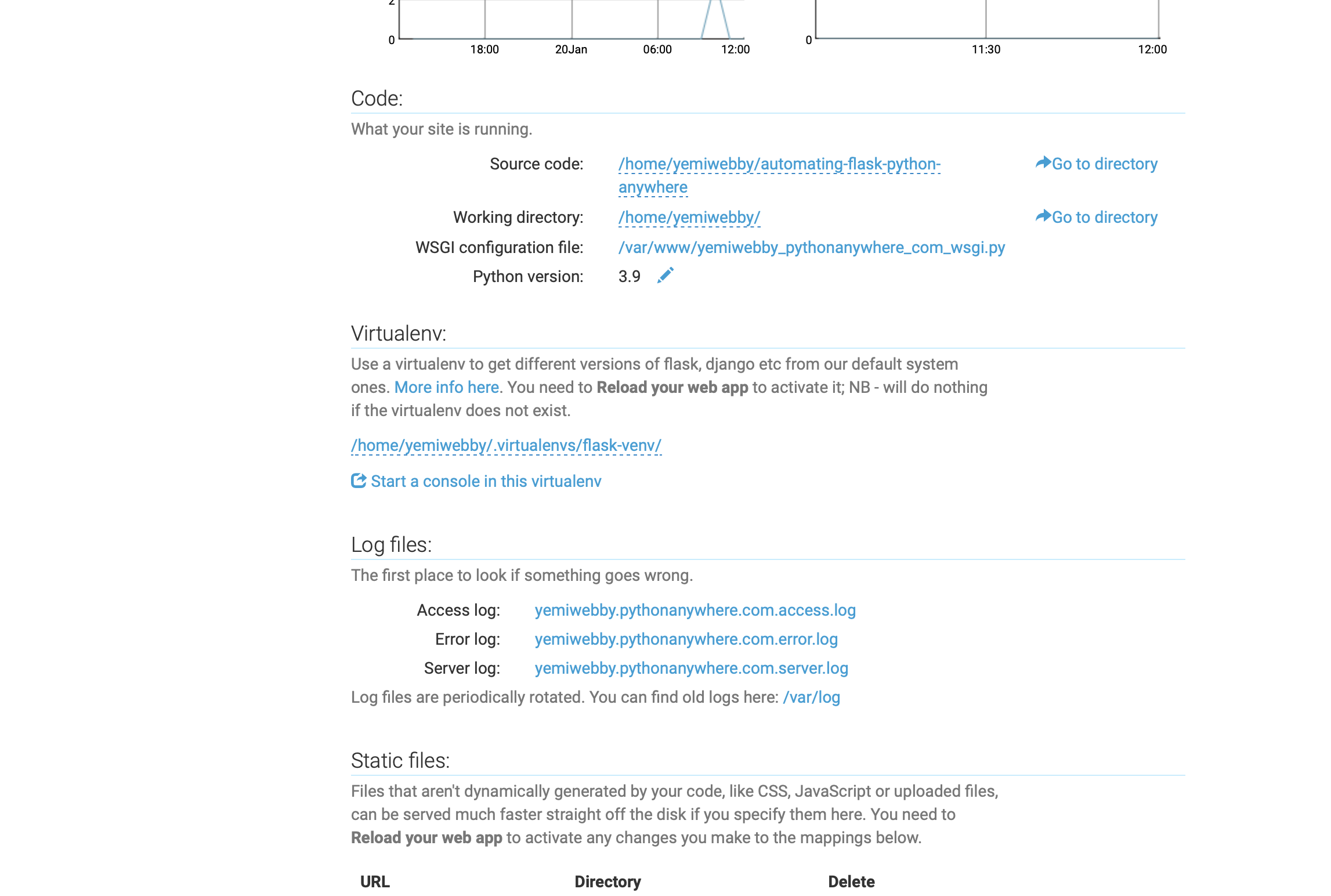At the top of the image, there are two horizontal lines with numbers beneath them, resembling a graph setup. The first line features the number "1808," while the second line is labeled with "20th January" and extends to "12 o'clock." 

Beneath this section, the word "Code" is prominently underlined with a long blue line. Below it, there is a label that reads "What your site is running." 

Further down, you'll find the heading "Source Code," followed by a clickable blue link positioned to the right. Adjacent to it is another heading labeled "Working Directory," accompanied by another interactive blue link, and below that, headings for "WSGI Configuration File" and "Python Version." Next to the Python Version label, it specifies "3.9" and displays the image of a blue pencil.

The subsequent section is titled "Virtual ENV," followed by a brief paragraph in bright blue text that reads "More info here." Below this, there is an option to "Start a console in this virtual ENV."

The final section is labeled "Log Files," which is also underlined in blue. It includes a note stating, "The first place to look if something goes wrong." Vertically beneath this heading, there are three options: "Access Log," "Error Log," and "Server Log."